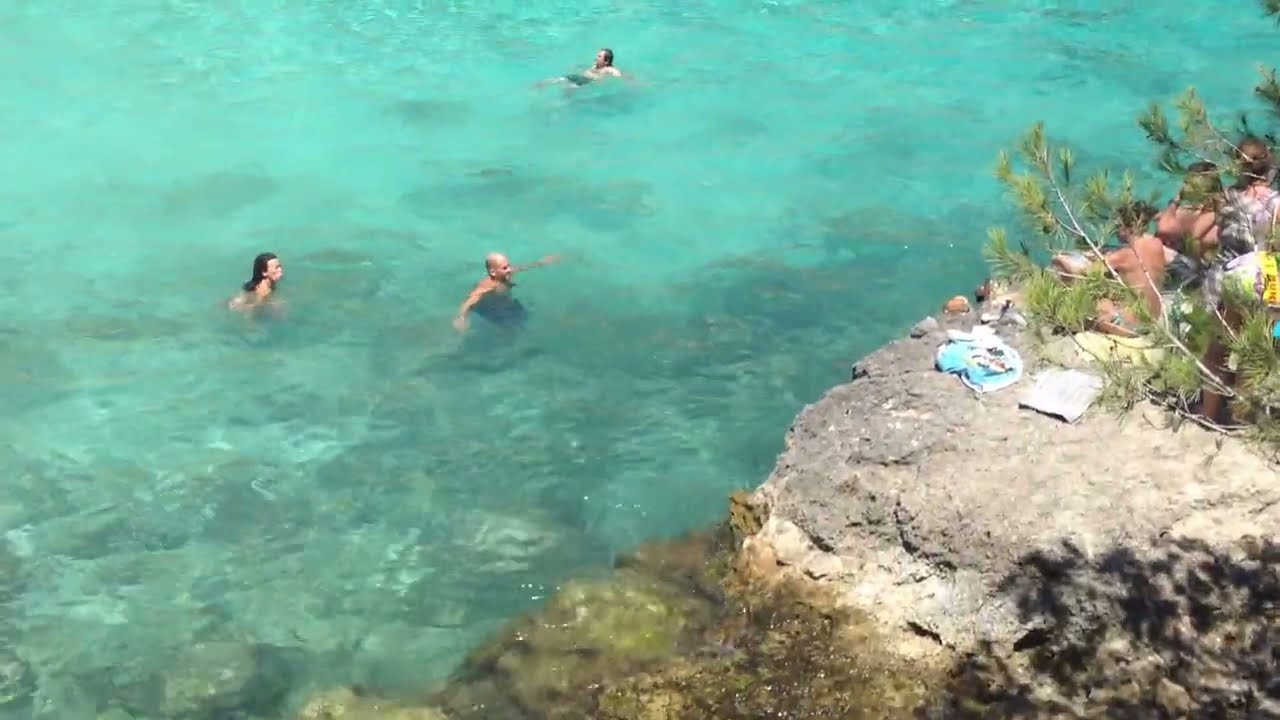In the overhead image, several people are seen swimming in a clear, shallow, aqua-blue to greenish body of water, revealing the brown rocks beneath. To the left, three individuals—a woman with shoulder-length black hair, a bald man extending his arms just below the surface, and another man floating on his back—are engaged in swimming. The water is transparent and pristine, offering a detailed view of the underwater landscape. On the right, adjacent to the swimmers, a large, flat, gray rock formation is present. Three women, seated on this rock, appear to be observing and interacting with the swimmers below. These women are distinctly dressed: one, closest to the viewer, wears a bikini, while another, further back, dons a full white dress. Partially obscuring the scene are tree branches with small leaves extending into the frame. The overall setting suggests a popular spot for cliff diving or casual swimming, with vibrant natural scenery including verdant plants and bushes surrounding the area.